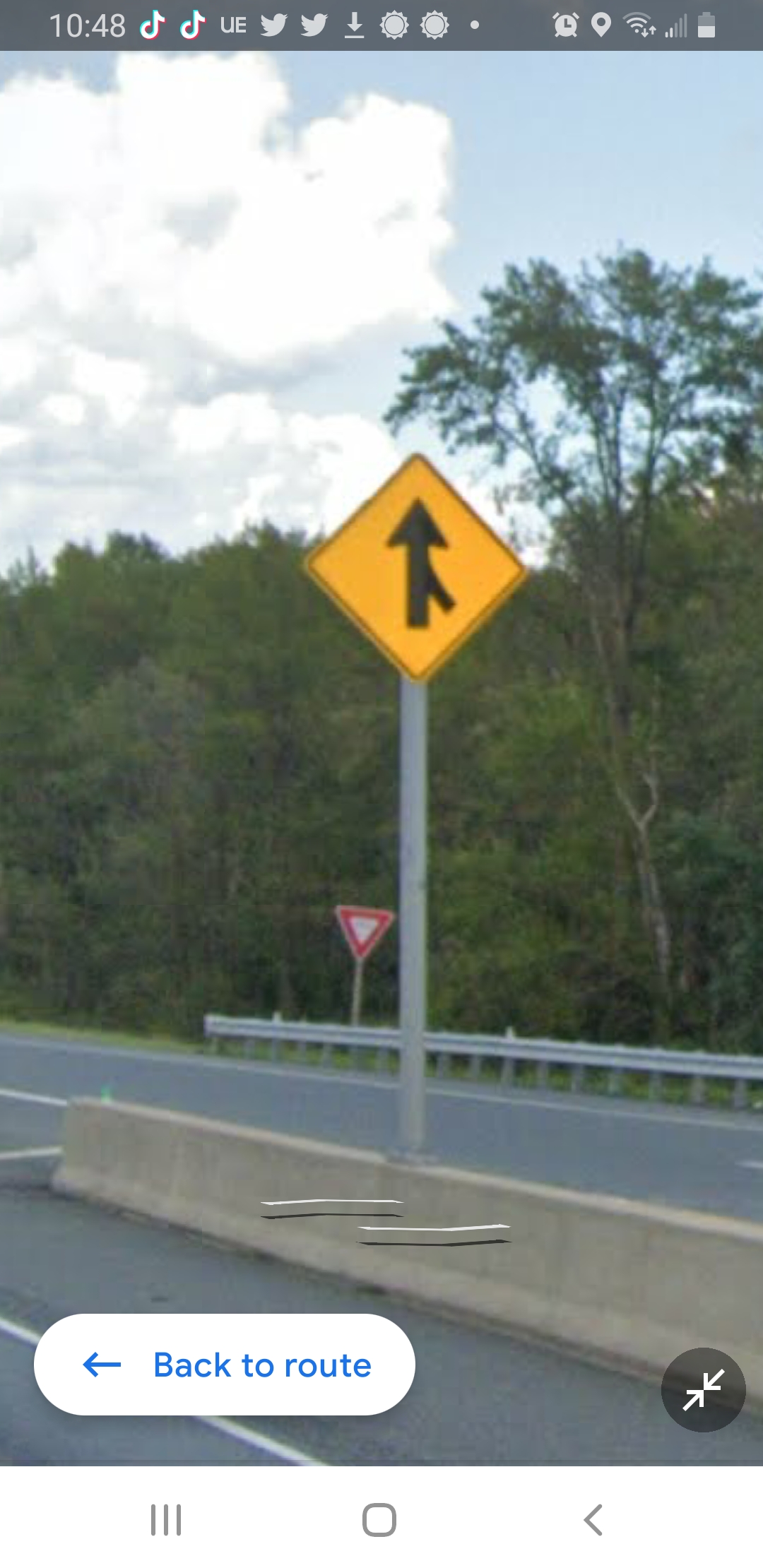This image is a detailed screenshot from a cell phone, likely a Google Street View capture. Dominating the scene is a road segment with visible highway pavement and white road lines. The sky's blue hue is tinged with fluffy white clouds. A dense assembly of trees, primarily boasting heavy green foliage, lines the scene, with one notable tree appearing bare. 

The central focus includes road signs; a prominent yellow diamond-shaped sign depicts a vertical arrow with a merging lane from the lower right, indicating an upcoming lane merge. This sign is mounted on a concrete barrier. In the background, there's a red and white triangular yield sign. A guardrail or steel border runs along the opposite side of the road, hinting at a possible bridge due to its straight, terminating structure. 

Overlaying the image are UI elements of the cell phone screen: the time displayed as 10:48, icons for various functions such as TikTok, UE, and Twitter apps, signal strength, battery status, and a navigation prompt with arrows indicating direction. These details collectively frame the roadway scene within the context of modern digital navigation tools.